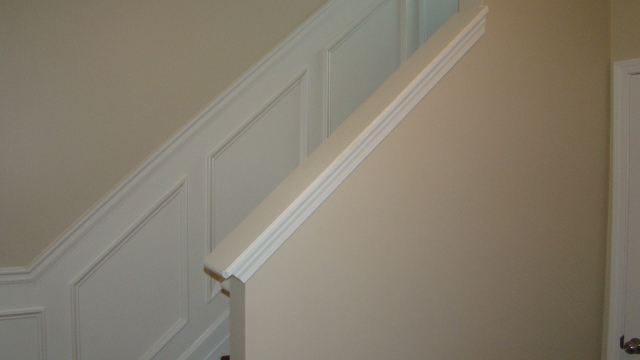This color photograph, taken indoors, likely within a residential home, depicts a staircase viewed from a side angle. The walls are painted in a hue that variously appears as brown, beige, or light rose, accompanied by decorative white trim at the bottom. The staircase features a handrail and intricate white paneling that ascends along with it, indicating its upward direction. At the bottom corner of the image, the trim is oriented horizontally, confirming this is the base of the staircase. The staircase itself appears to be made of dark wood. On the right side of the photograph, a white door with a silver doorknob is visible, suggesting an adjoining room. The overall setting seems to be an entryway or foyer of the house.